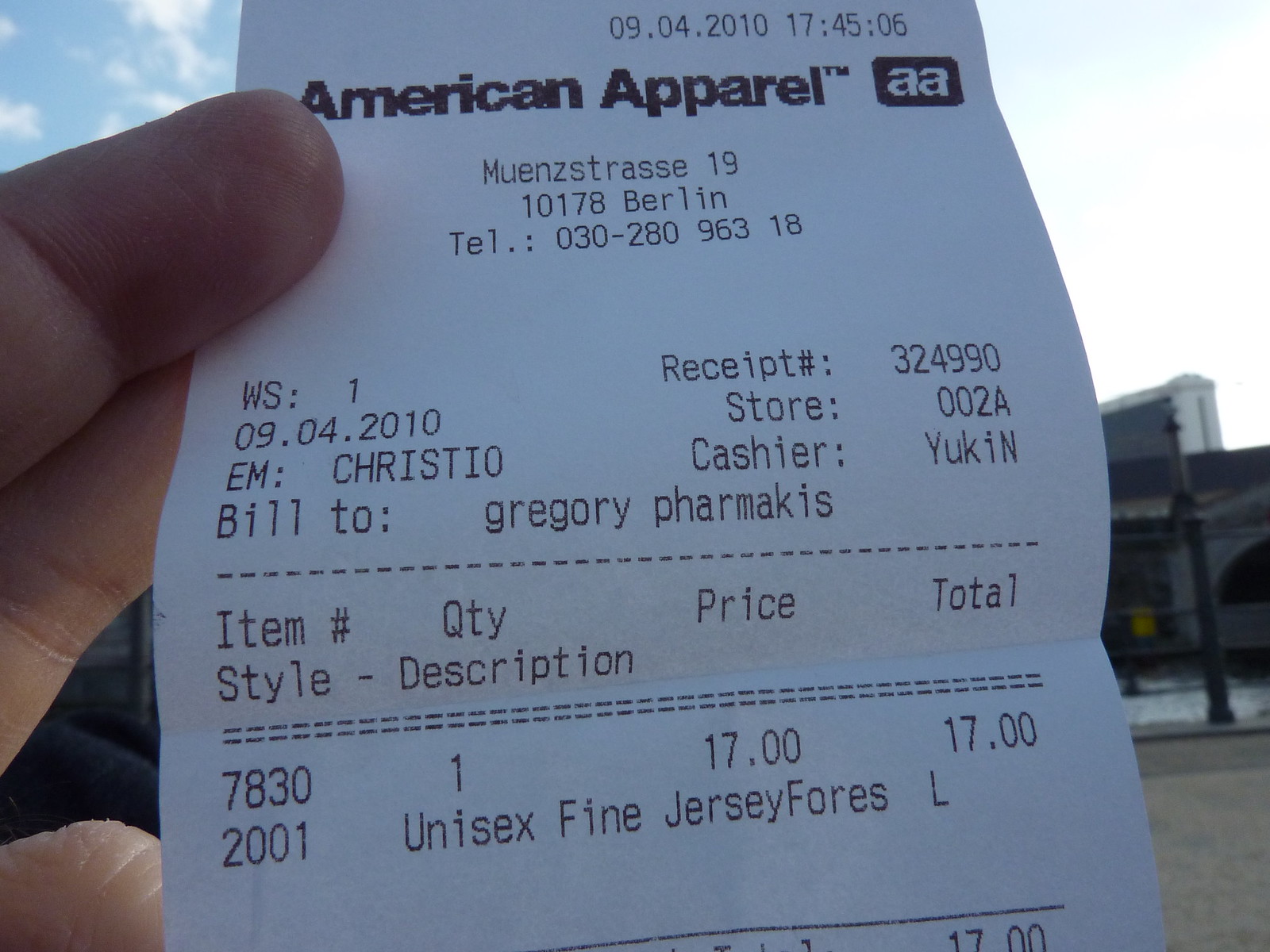A photo depicts a person's left hand holding a white, rectangular receipt between their index and middle fingers. The receipt is from American Apparel in Berlin, printed in bold black ink at the top. The date "09.04.2010" and the time "17:45:06" are stamped across the top. The receipt details include the name "Gregory Farmacchi" as the billed individual and the cashier’s name, "Yukin." The purchase made was for one unisex fine jersey, costing $17.00. In the background, there is a blue sky with white clouds and a building. The right corner of the image shows a blurred sign, while the left side prominently features the hand holding the receipt.